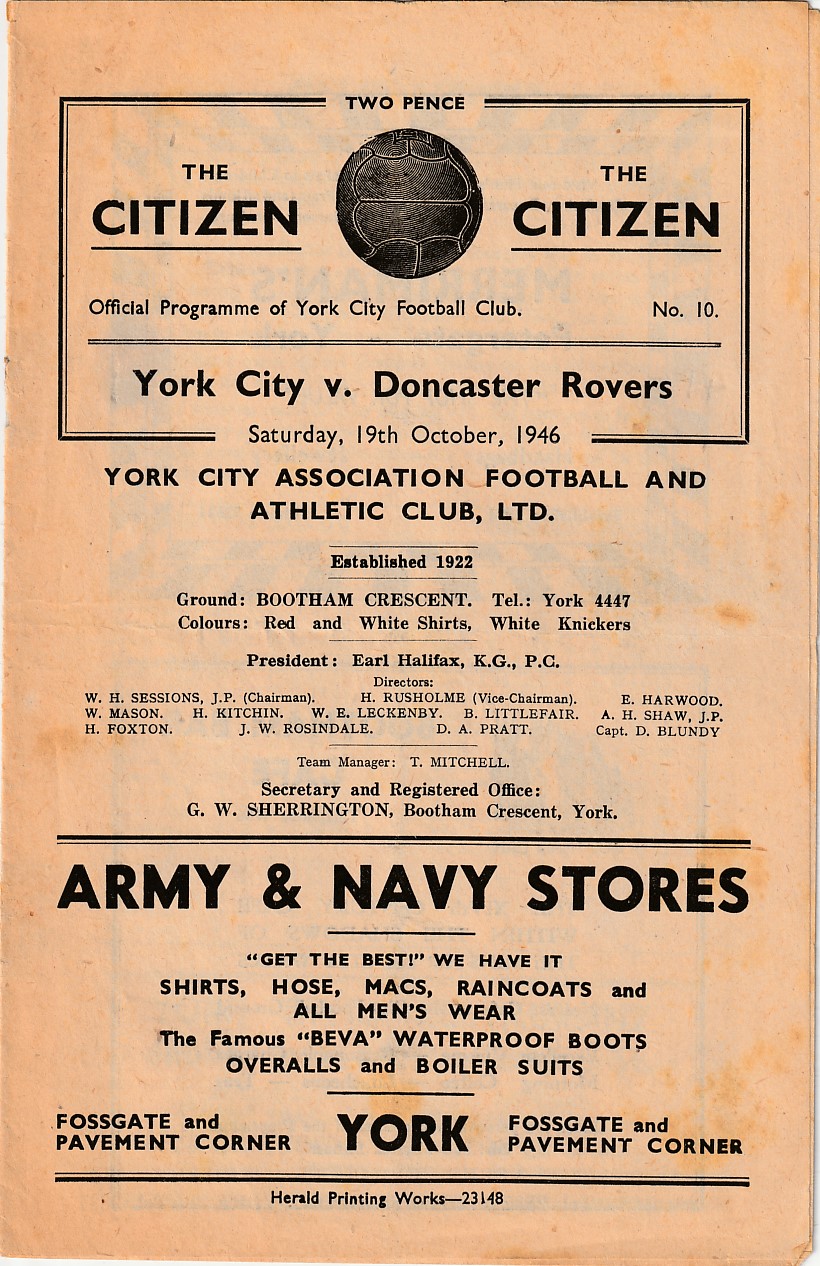The image features a weathered off-white pamphlet with black lettering. At the top, there is a box with the text "Two Pence." Inside the box, a soccer ball is centered, flanked by the text "The Citizen" on both sides. Below the soccer ball, it reads "Official Program of New York City Football Club, Number 10." A line separates this from the larger text, which states "New York City vs. Doncaster Rovers, Saturday, 19th October 1946."

Below the box, the text continues with "New York City Association Football and Athletic Club, LTD," followed by "Established 1922." The text lists pertinent details such as the club's ground at Bootham Crescent, the contact telephone number York 4447, and the team colors: red and white shirts with white knickers. The President is Earl Halifax, KGPC.

The pamphlet also lists the club's personnel:
- Directors: W.H. Sessions, J.P. (Chairman), W. Mason, H. Kitchen, H. Foxton, J.W. Rosdell, H. Rossholm (Vice Chairman), W.E. Lickenby, B. Littlefair, D.A. Pratt, E. Harwood, A.H. Shaw, J.P.
- Captain: D. Blundy
- Team Manager: T. Mitchell
- Secretary and Registered Office: G.W. Sherrington, Bootham Crescent, York

An advertisement at the bottom section of the pamphlet promotes "Army and Navy Stores" with the slogan: "Get the Best, We Have It." The ad lists products such as shirts, hose, macs, raincoats, and all men's wear, as well as the famous Belva waterproof boots, overalls, and boiler suits. The store location is cited as Fosgate and Pavement Corner, York. The pamphlet concludes with "Harold Printing Works, 23148."